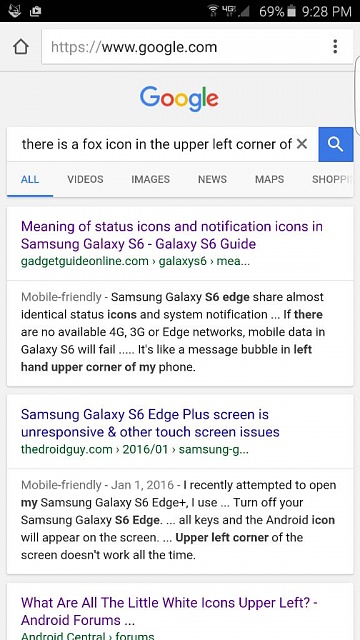The image depicts a cell phone screen displaying a website from Google. It is currently 9:28 PM, and the battery life is at 69%, with the phone operating on a 4G network. In the upper left corner, there are two icons present, while a black bar extends across the top of the screen. Below this bar is a search bar with the URL www.google.com, alongside a home icon and three vertical dots on the right side.

The Google logo is prominently displayed in its characteristic blue, red, yellow, and green colors. Directly beneath the logo, there is a fox icon and an "X" in the upper left corner, followed by the search icon within a blue box. The search bar also features a blue underline to indicate an active state.

The search results highlight a specific link titled "Meaning of status icons and notification icons in Samsung Galaxy S6—Galaxy S6 Guide" from the website gadgetguideonline.com, displayed in green text. Beneath this, a snippet indicates that the article is mobile-friendly and discusses the nearly identical status icons and system notifications of the Samsung Galaxy S6 Edge. The subsequent result pertains to troubleshooting the unresponsive screen and other touchscreen issues with the Samsung Galaxy S6 Edge Plus. This link is marked as mobile-friendly and is followed by a purple link titled "What are the little white icons upper left" from Android forums.